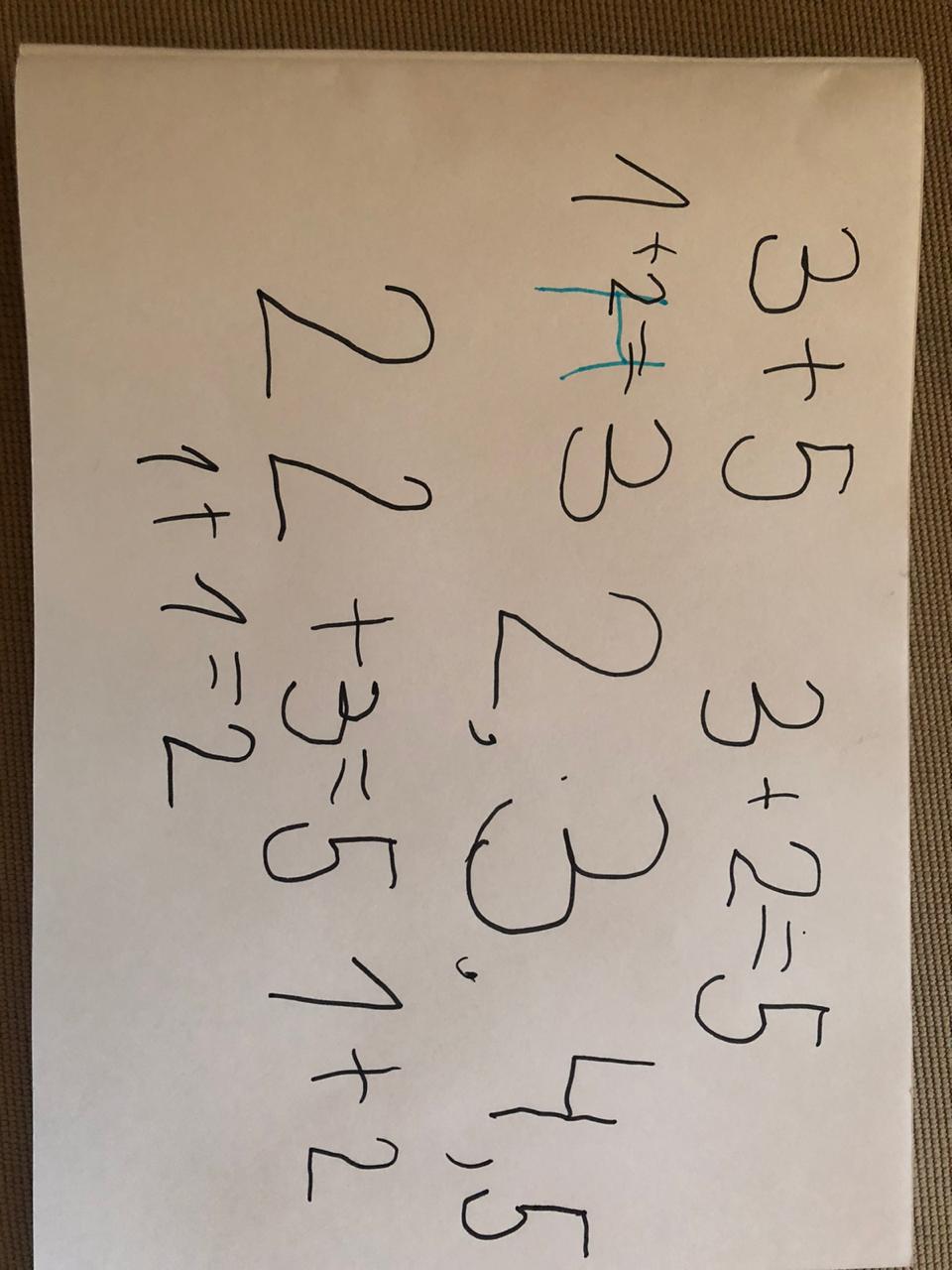The photograph showcases a piece of paper resting on a table. The table surface visible from the upper right to the lower right of the image reveals a tightly woven, knitted fabric with shades of orange and red, resembling a carpet. Upon closer inspection, one can see a crease along the top left to the right edge of the paper, suggesting that the paper may be part of a notebook or notepad and has been slightly rolled back.

The paper itself, viewed from its side, contains a series of handwritten mathematical equations. Starting from the top left corner, the first equation reads "3 + 5," followed by "3 + 2 = 5." Below these equations, there is an incorrect statement, "7 + 2 = 3," which is marked with a large blue "H" likely indicating an error. Beneath this, a series of numbers "2, 3, 4, 5" is listed sequentially. The third row contains another incorrect equation, "22 + 3 = 5," and the subsequent line states "7 + 2."

The final row features yet another incorrect equation, "7 + 7 = 2," where the numeral "1" might have been mistaken for a "7." Returning to the top right corner, there is the equation "1 + 2 = 3," marked with blue ink. The bottom left corner again shows a similar mix-up where "1 + 2" appears with the numeral "1" written in a manner that resembles a "7." The last equations state "1 + 1 = 2."

Overall, this detailed visual document appears to be a combination of both correct and incorrect simple arithmetic equations, some of which have been highlighted with blue ink for correction.